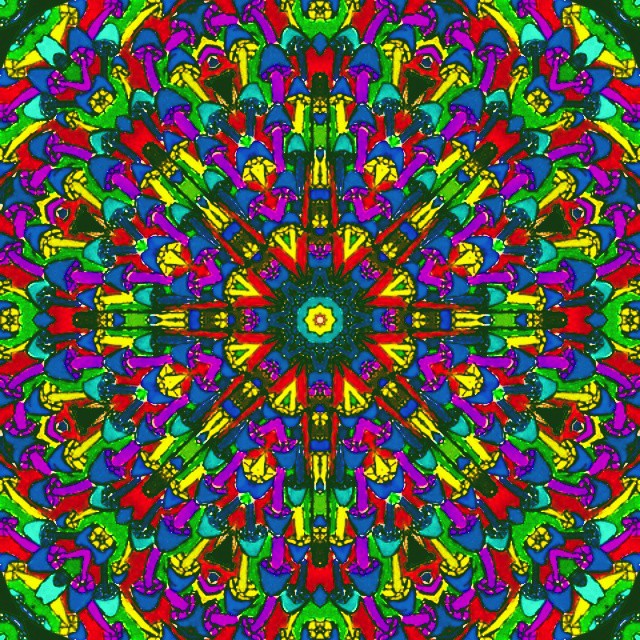The image showcases a vibrant and intricate piece of graphic art with a psychedelic flair. At the center, there's a detailed emblem in red and yellow, encased in a square. This centerpiece is surrounded by an octagon which is further encompassed by a green band, followed by a dark blue band. There’s also a band of yellow and green triangles with their points directed towards the center. Radiating from this central emblem are eight arms extending in all primary and diagonal directions.

Encircling these central elements, there are concentric patterns featuring red, blue, and purple mushroom-shaped motifs. The overall design resembles a kaleidoscope or mandala, with a central yellow blossom pattern stemmed by green mandala outlines, progressing outward into blue offshoots. Red and yellow V shapes with central green dots are prominent, succeeded by layers in magenta, yellow, blue, turquoise, red, and green, creating an elaborate border.

This psychedelic image further incorporates various shapes—triangles, octagons, stars, and half-moons—meticulously arranged to form a comprehensive and harmonious circular pattern. The use of diverse and vivid colors like fluorescent green, teal, purple, red, yellow, and light blue, all contribute to the mesmerizing and intricate composition of this artwork.